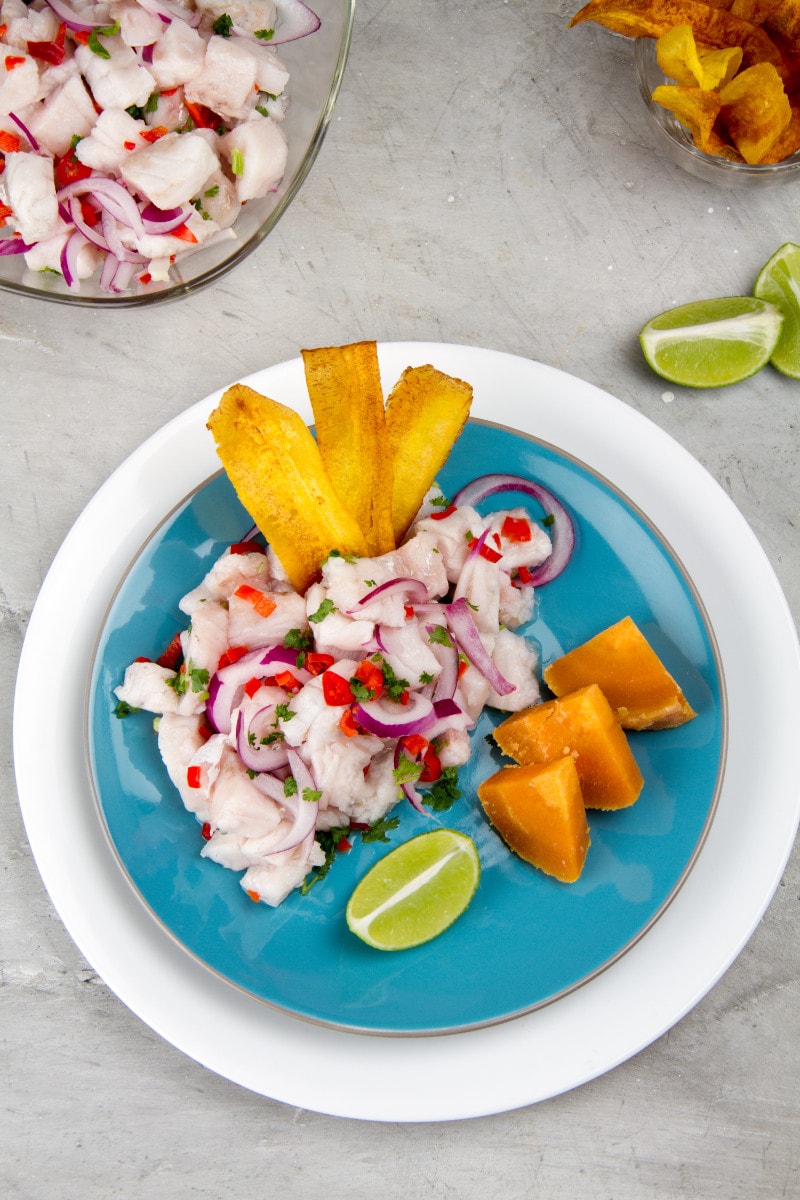The photograph is a vertically aligned rectangular image measuring approximately 6 inches tall by 4 inches wide, taken from a top-down perspective. It showcases a selection of food items arranged on a gray, marble-like granite countertop featuring light and dark gray streaks. Dominating the center of the image is a large white plate, partially extending out of the frame on the right. Positioned atop the white plate is a slightly smaller blue plate with a gold rim, highlighting the focal dish, which appears to be a ceviche composed of white fish, mixed with red onions, red chilies, and herbs. The ceviche is garnished with three rectangular fried plantain chips and a slice of lime. Accompanying the ceviche on the blue plate are three triangular wedges, possibly sweet potatoes or fermented ginger. 

In the upper left corner of the image, a clear glass bowl contains more of the white fish ceviche with red onions. The upper right corner features another clear glass bowl filled with what appear to be potato crisps or fried plantains. Below this bowl are a couple of lime slices resting directly on the countertop. The overall setup captures an intricate and colorful presentation of the ceviche dish and its accompaniments on a beautifully textured gray marble surface.